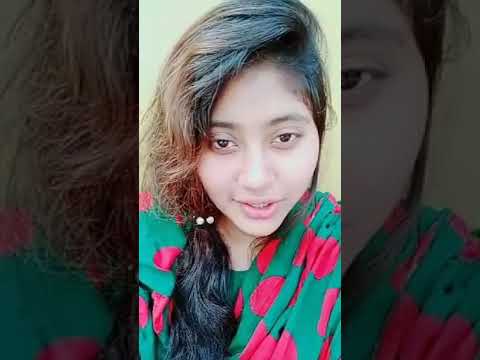The image features a young girl with medium to light skin and mid-length to long dark brown hair that has two tones—darker brown in the middle and lighter brown on the side. Her hair is pulled into a deep side-part ponytail that falls over her right shoulder and is adorned with a couple of beads. She looks downward with her eyes slightly upcast toward the camera, giving the impression that she might have taken the photo herself. She appears to be wearing very light pink lipstick.

Her attire is a green shirt, possibly a blouse or jacket, adorned with a red or pink design, described variably as splotches or large polka dots. The background of the image includes light tan or yellowish walls, and the photograph is framed with black rectangles on either side, giving it a landscape orientation despite originating as a portrait. The overall image has been edited to include a more zoomed-in version overlaid with a dark filter. The dimensions of the full image are approximately five inches wide by four inches tall, without any additional text or other images.